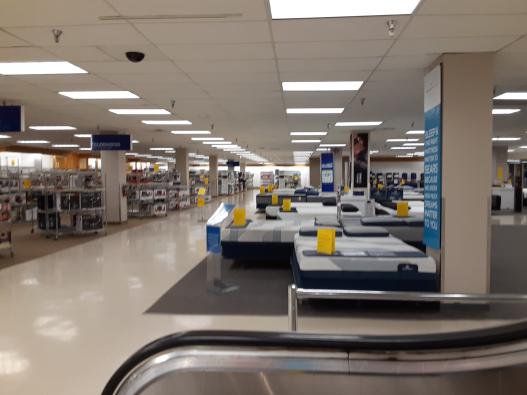This image captures the interior of a retail store, prominently featuring an escalator in the center, ascending to the next floor. Behind the escalator, the sales floor is visible, specifically the bedding section, where various beds are displayed in a minimalist manner for customers to test. Each bed features a yellow price tag. To the left of the beds, the home goods department is partially visible. The store’s architecture includes multiple columns supporting the ceiling, all equipped with sprinkler systems for safety. In the top left corner of the image, there is a black dome concealing a security camera, ensuring the store is under surveillance.